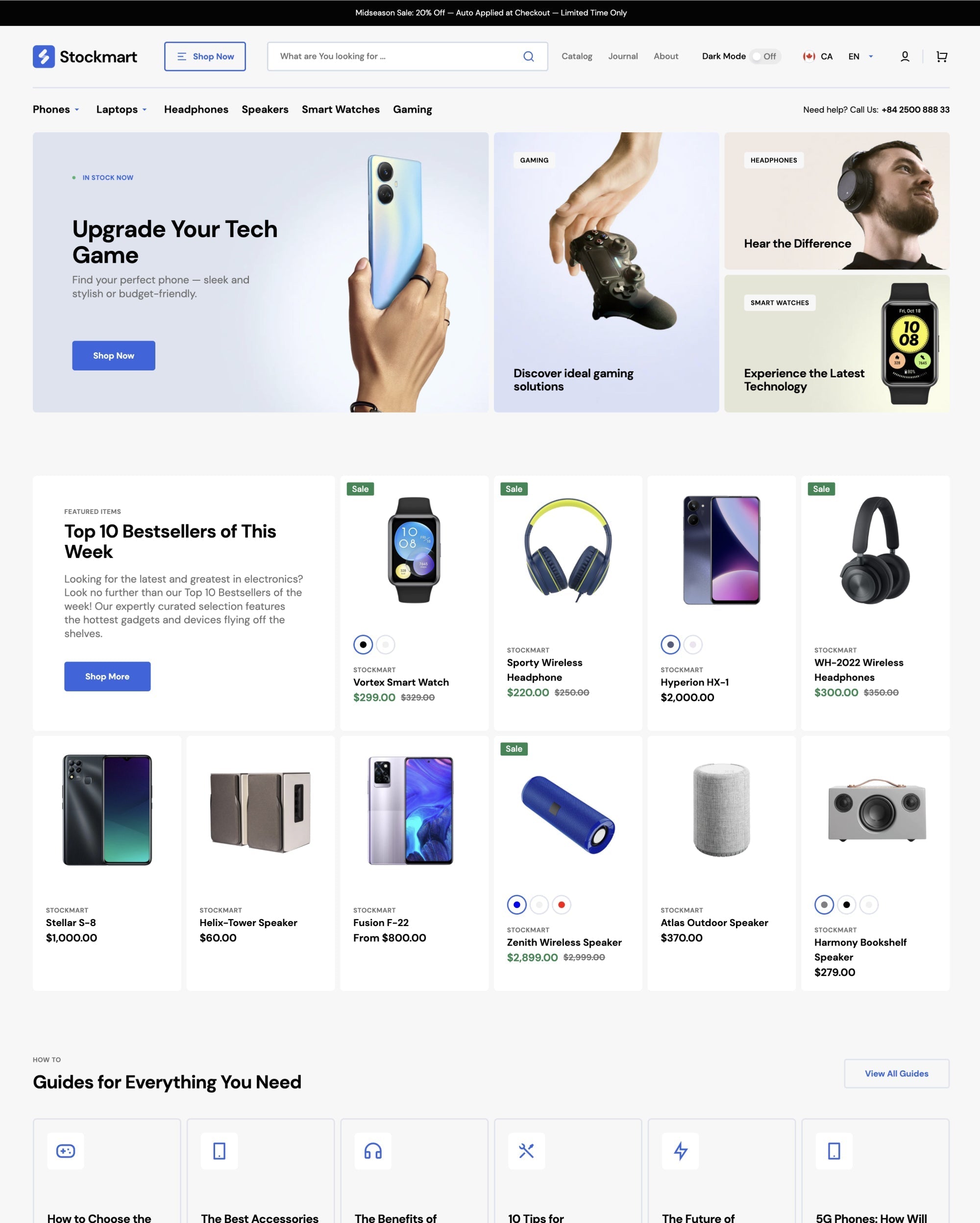This is a detailed view of the homepage for the shopping website Stockmart, S-T-O-C-K-M-A-R-T. At the top of the page, a prominent advertisement banner reads, "Upgrade your tech game, shop now," urging visitors to elevate their technology with immediate purchases. Adjacent to this headline is a callout, "Discover Ideal Gaming Solutions," accompanied by an image of a gaming controller. Following this, the next two promotional boxes to the right feature catchy taglines: one promotes headphones with "Hear the Difference," highlighting a focus on audio quality, and another showcases a smartwatch with the caption "Experience the Latest Technology," emphasizing cutting-edge advancements.

Below the promotional banners, the main section features a headline announcing the "Top Ten Best Sellers of This Week," showcasing the site's most popular products. The top ten bestsellers include:

1. Vortex Smart Watch
2. Sporty Wireless Headphones
3. Hyperion X1 Smart Phone
4. WH-2220 Wireless Headphones
5. Stellar S8 Smart Phone
6. Helix Tower Speaker
7. Fusion F22 Smart Phone
8. Zenith Wireless Speaker
9. Atlas Outdoor Speaker
10. Harmony Bookshelf Speaker

This detailed overview of Stockmart's homepage emphasizes its diverse range of electronic items, suggesting that it caters to a wide array of tech needs, from smartphones and wearables to high-quality audio solutions and gaming devices.